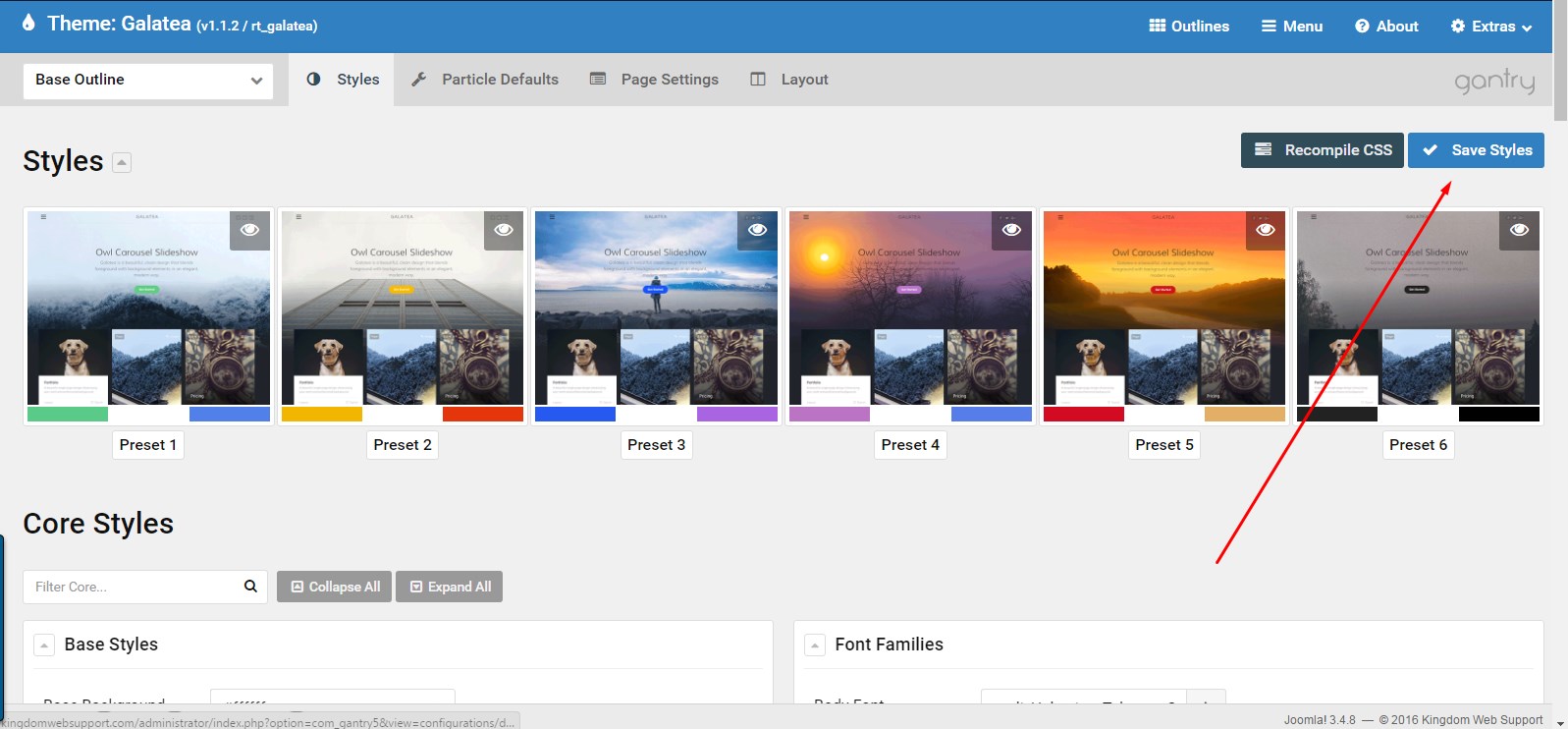The image features a rectangular interface with a blue banner at the top. The banner includes a white font heading that reads "Theme: Galatea." To the right of this heading, there are menu options labeled "Outlines," "Menu," "About," and "Extras," each with a drop-down menu.

Below the banner, there's a white search box with a drop-down menu displaying "Base Outline." Adjacent to this on the right, there are gray tabs with black text labeled "Styles," "Particle Defaults," "Page Settings," "Layout," and "Gantry."

Underneath these elements, a lighter gray bar with black text indicates another drop-down menu titled "Styles." Following this, there are six template images labeled "Preset 1," "Preset 2," "Preset 3," "Preset 4," "Preset 5," and "Preset 6," intended for use in content creation.